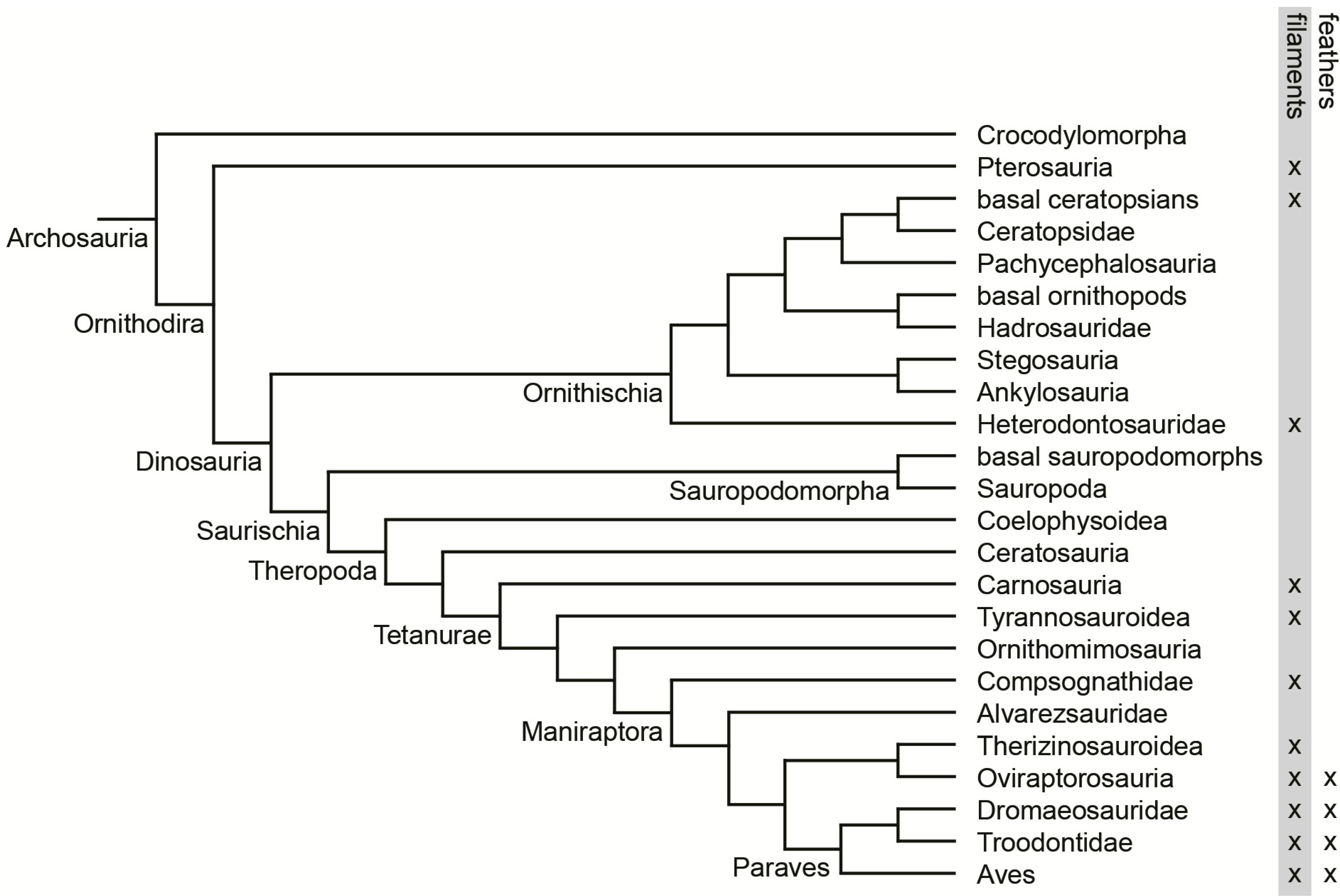The image is a black-and-white chart resembling a tournament bracket or a tree diagram, but it's actually a classification chart of various dinosaur categories. Starting on the left, there are eight primary categories: Archosauria, Ornithodira, Dinosauria, Saurischia, Theropoda, Titanura, Maniraptora, and Paraves. From each of these categories, lines branch out to additional names such as Stegosaurus, Ceratosauria, and Tyrannosaurus, indicating a hierarchical relationship. On the far right of the chart, there are two vertical bands—one labeled "feathers" in black text on white and the other "filaments" in black text on gray. X's mark which dinosaurs had feathers or filaments. Despite the detailed arrangement, the chart has no title to clearly indicate its subject matter, relying instead on the reader’s interpretation of the terms and the structure.